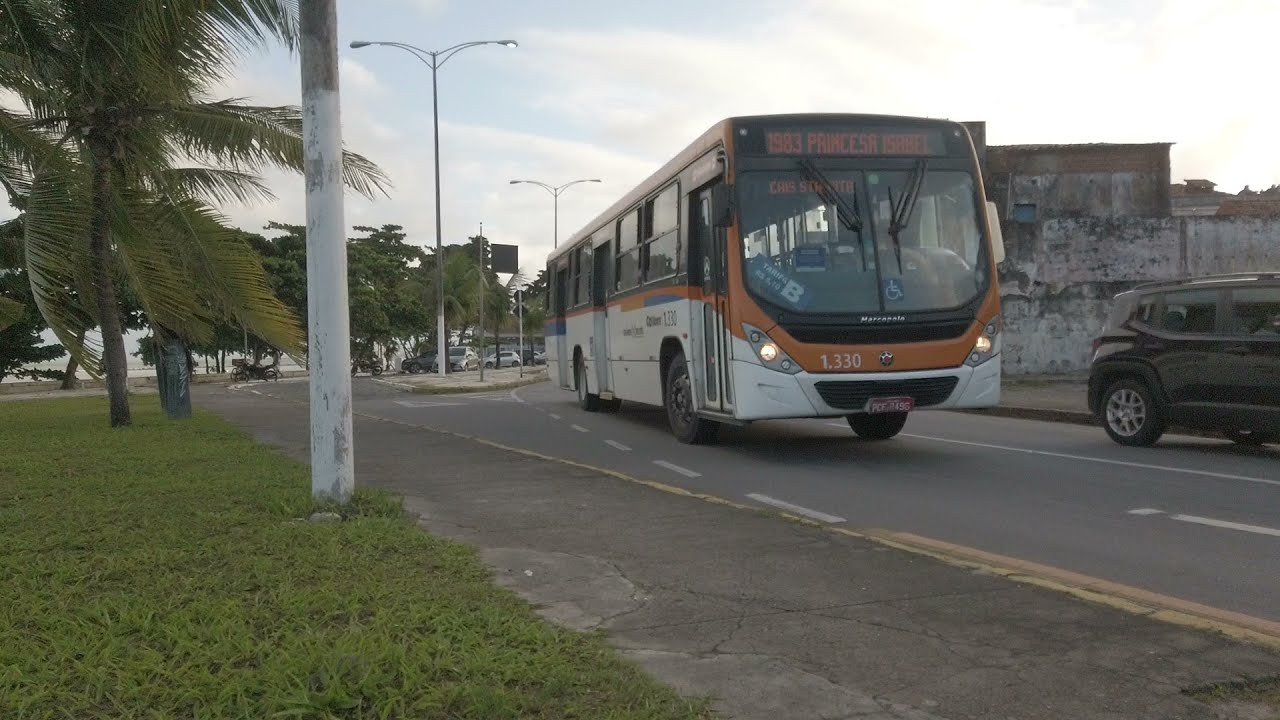In the center of the image, a white and orange public bus marked "1983 Princesa Isabel" traverses a busy urban road. The bus's headlights are on, and visible on its front are the numbers 1330 and a handicap symbol. To the right of the bus, partially cut off, is a black, boxy, four-door car resembling a Scion. Both vehicles are framed by a gray and tan building in the background, with noticeable chipping paint and a worn, industrial look. To the left of the road is a sidewalk that borders a grassy area adorned with several palm trees and multiple white-painted street lights, though some poles are cropped by the image's edge. The scene is bathed in daylight under a light blue sky sprinkled with white clouds.